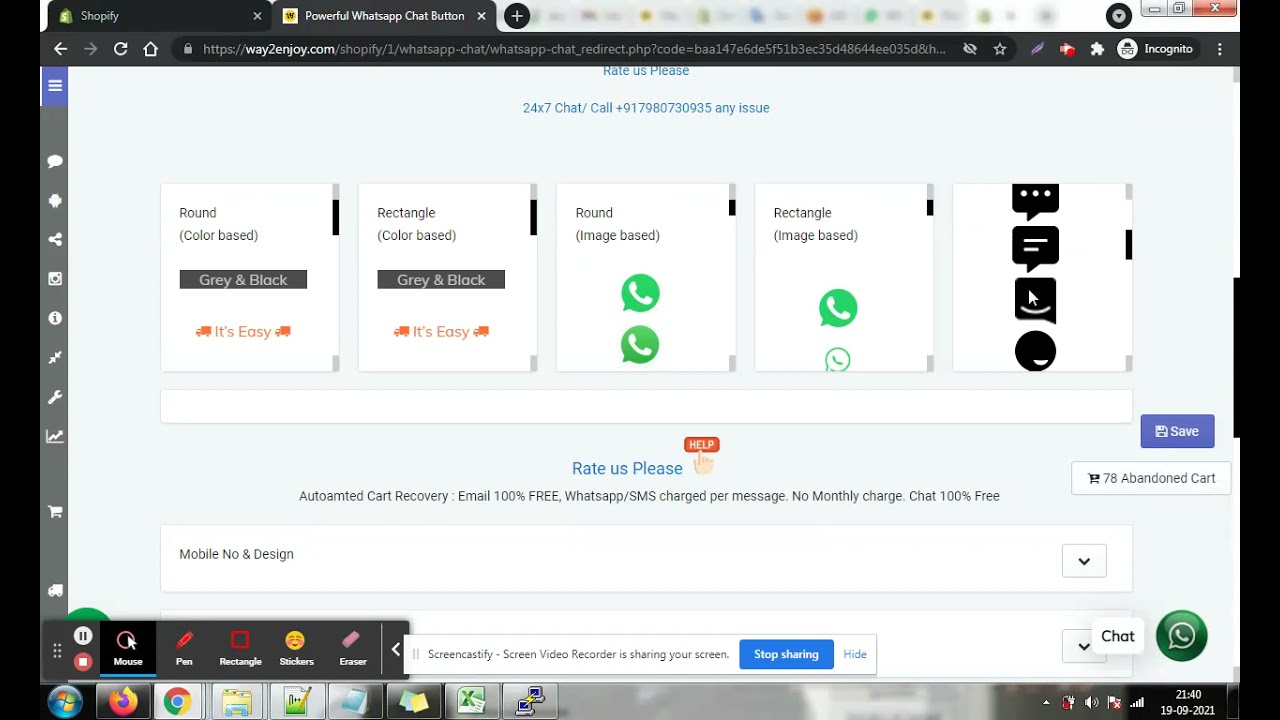A detailed screenshot capture of a web browser displaying two active tabs at the top: one for Shopify and another for a WhatsApp chat window. The currently active tab is the WhatsApp chat, highlighted. Below the tab bar, the main screen displays a settings menu for WhatsApp chat customization. In the settings interface, there are five square menu tiles arranged on the screen. Each tile is labeled according to its shape preferences: two are labeled "Round", two are labeled "Rectangle", and one more is also labeled "Round". These options appear to let users configure the display shape preferences for their WhatsApp chat interface.